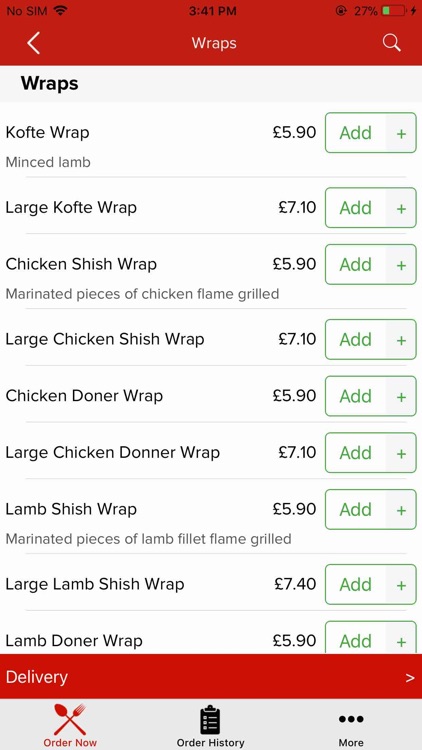The image depicts a section from a food or delivery app, specifically focusing on a variety of wraps accompanied by their prices in British pounds. The section is titled "Wraps" and includes several options such as Kofte (minced lamb), Chicken Shish (marinated pieces of chicken flame-grilled), Chicken Doner, Lamb Shish (marinated pieces of lamb fillet flame-grilled), and Lamb Doner. The prices for these wraps range from £5.90 to £7.10. Each wrap option has an "Add" button to the right, allowing users to easily add items to their order. At the bottom of the screen, there are three navigation tabs: Order Now, Order History, and More. The app's interface features a predominantly white background with some red elements for visual contrast. A back button is also visible, presumably allowing users to return to the larger menu.